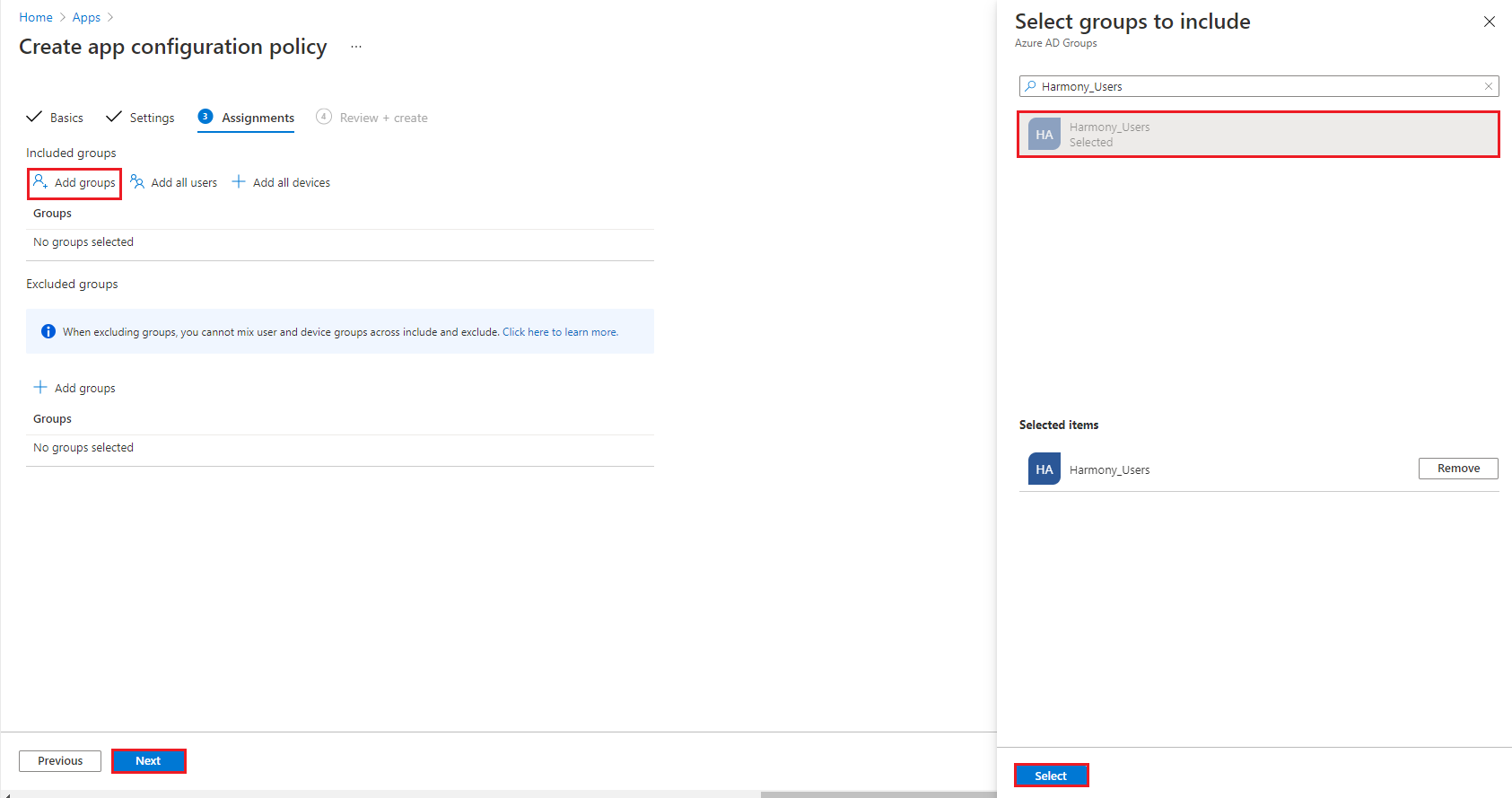The image is a screenshot of a web page displaying app configuration settings. The layout is divided into two main sections. The left section occupies approximately two-thirds of the screen, while the right section takes up the remaining third.

### Left Section
- **Header Navigation**: 
  - At the top left, in blue text, it reads "Home > Apps > Create App Configuration Policy," with arrows pointing to the right between the terms.
  
- **Title and Menu**:
  - Below this navigation, the title "Create App Configuration Policy" is prominently displayed in large black text. To the right of the title is a button with three dots.

- **Progress Steps**:
  - Several sections are listed vertically:
    - "✔ Basics"
    - "✔ Settings"
    - "3 Assignments" (highlighted in blue, indicating the current section, with a blue circle containing the number three, underlined in blue)
    - "4 Review + Create" (grayed out, indicating it is not yet active)

- **Assignment Options**:
  - Under the "Assignments" section, the subheading "Included Groups" is displayed.
  - Three buttons are available: "Add Groups," "Add All Users," and "Add All Devices."
  - A thin gray line separates this section from the term "No Groups Selected."
  - Another darker gray line separates it from the next subheading, "Excluded Groups."

- **Exclusion Options**:
  - Beneath "Excluded Groups," there is a light blue text box containing a message: "When excluding groups, you cannot mix user and device groups across Include and Exclude. Click here to learn more." The phrase "Click here to learn more" is in blue, indicating a hyperlink.
  - Below this, there is a blue plus (+) button labeled "Add Groups."
  - Further down, the text "Groups," followed by another thin light gray line and the term "No Groups Selected" beneath it.
  - Another darker gray line appears under these elements.

- **Navigation Buttons**:
  - At the bottom left of the screen, there are two navigation buttons: a white "Previous" button and a blue "Next" button.

### Right Section
- **Select Groups**:
  - The right third of the screen features a white background with the header "Select Groups to Include, Azure AD Groups."

This layout provides a clear and detailed view of the steps and options involved in creating an app configuration policy, with distinct sections for included and excluded groups, and intuitive navigation aids.